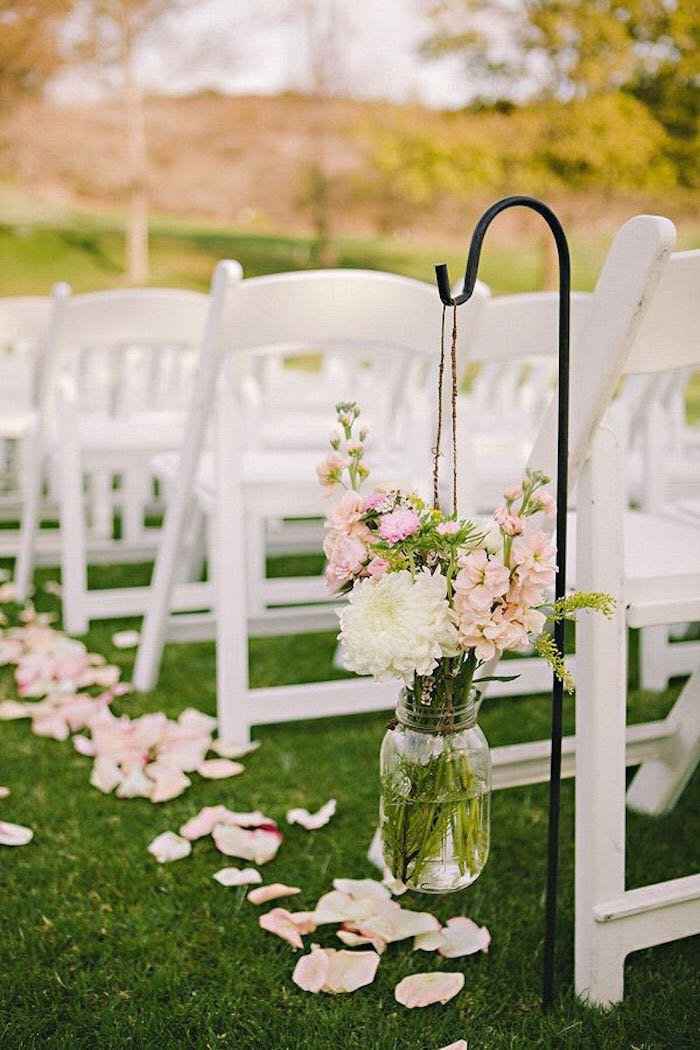The image captures a serene outdoor wedding venue under a bright blue sky with large green trees in the background. Rows of white chairs are aligned on lush, well-manicured grass, facing the front of the ceremony area. Scattered along the aisle beside the chairs are delicate pink and white flower petals. A black shepherd's hook stands prominently at the end of the closest row, elegantly curving at the top. Hanging from the hook by a brown string or twine is an old-fashioned mason jar, filled with water and a vibrant bouquet of wildflowers, featuring white peonies and pink lupines with green leaves. This mason jar arrangement mirrors the flower petals scattered on the ground, adding to the cohesive, rustic charm of the setting. The overall scene is bright and clear, enhanced by natural lighting that highlights the details beautifully.